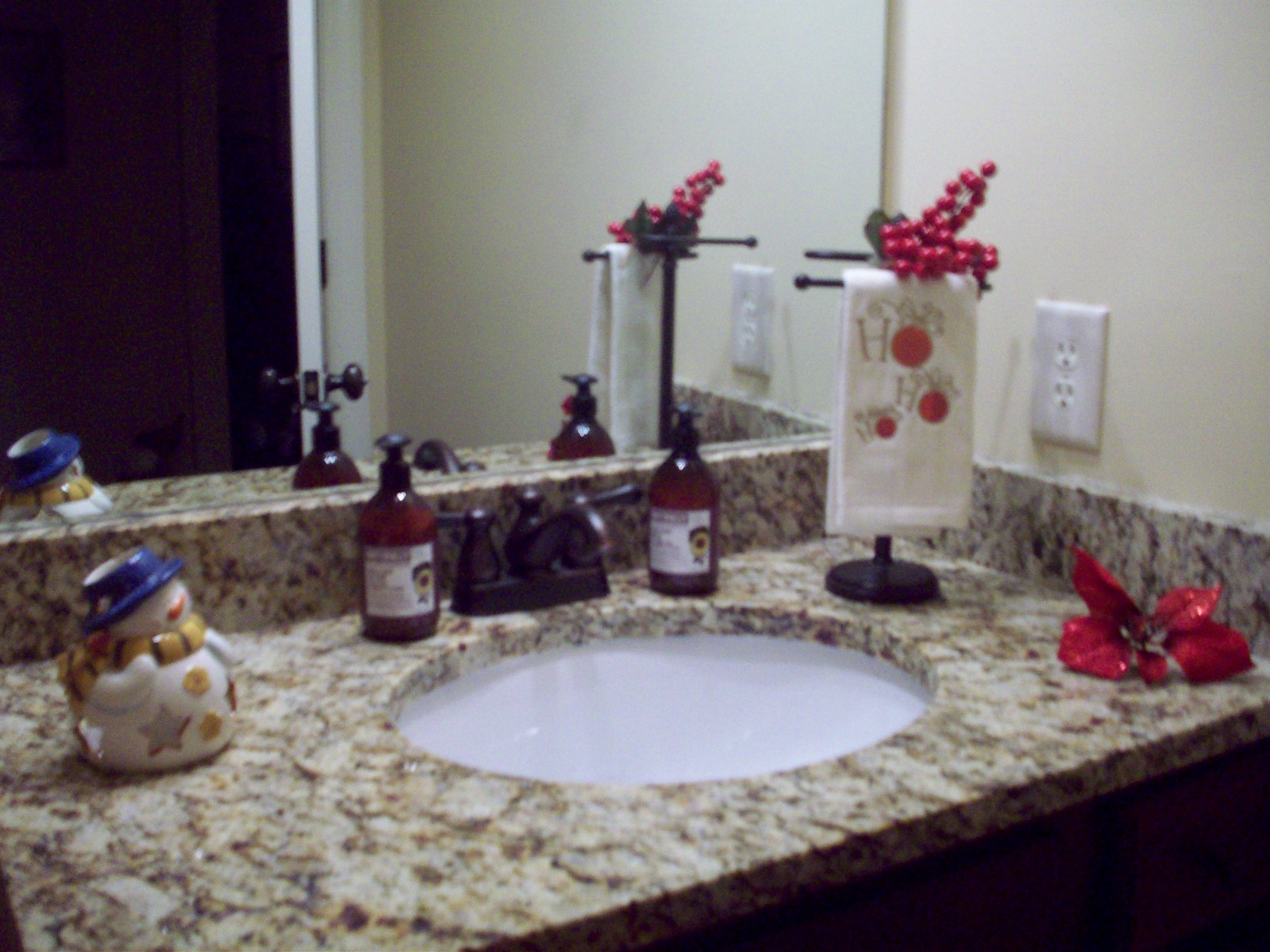The photograph depicts a cozy, homey bathroom adorned with festive Christmas decorations. The visible portion of the bathroom includes a counter, sink, and the mirror above the counter. The counter is made of a yellowish-white marble pattern, and it features a white sink bowl. On either side of the faucet, there are brown bottles with pumps and labels, likely containing soap and lotion.

To the left of the sink, a charming ceramic snowman candle holder or wax melter adds to the festive decor. The snowman is adorned with a blue hat, yellow scarf, and yellow buttons, with star cutouts on either side of the buttons. To the right of the sink, a metal towel holder is precariously balanced, holding a Christmassy towel that reads "HO HO HO" with red ornament-like 'O's. The towel holder is topped with decorative holly. Adjacent to the towel holder, an outlet is visible on the wall.

Adding a pop of color to the scene, a fake red sparkly poinsettia flower is placed on the counter. Reflected in the mirror is the open bathroom door, painted a clean white, completing this snapshot of a festive and inviting personal space.